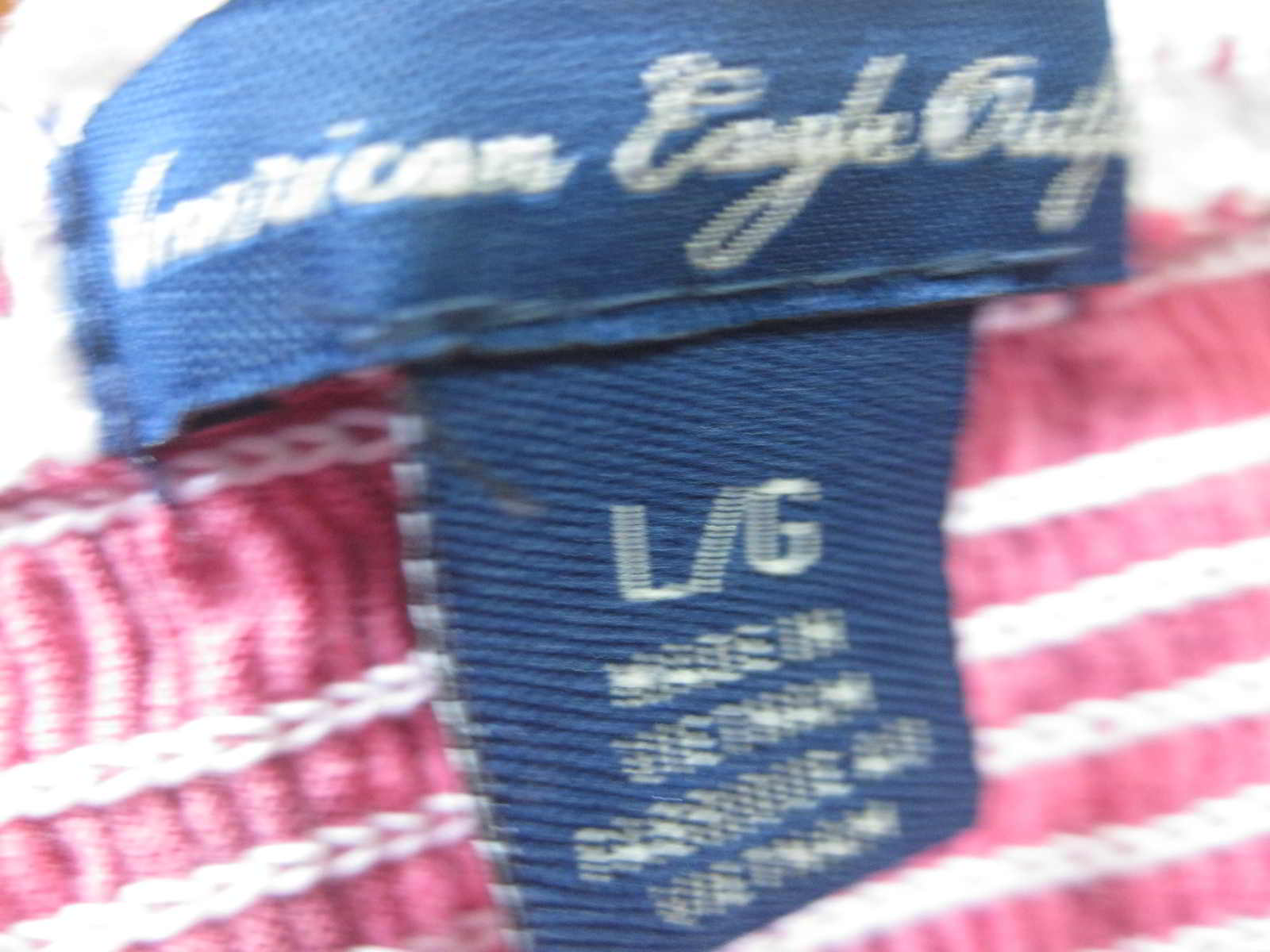A slightly blurred photo captures the inside tag of a piece of clothing. The visible portion of the garment is red with vertical white stitching. The tag is made of blue fabric and, although blurry, displays the partly obscured text "American Eagle Outfitters" curving around the inner collar seam. Beneath this primary label, a secondary tag indicates the size as "L/G" for large and includes the text "Made in Vietnam," followed by a translation in smaller, harder-to-read text.